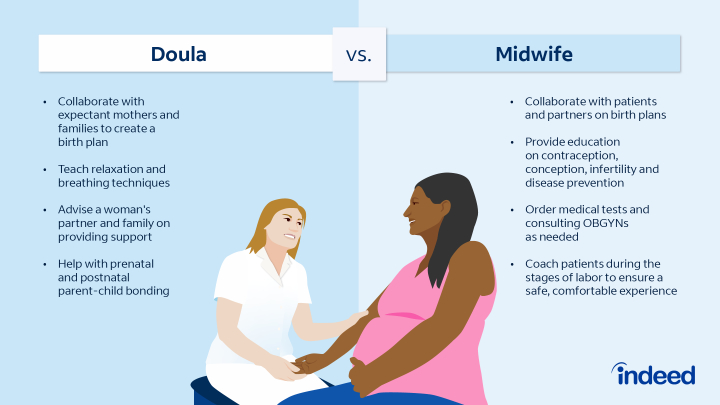The image is a comparison chart titled "Doula vs. Midwife," showcasing the roles and responsibilities of each profession. The chart is split into two sections: a dark blue section on the left labeled "Doula" and a light blue section on the right labeled "Midwife." 

Under "Doula," the chart bullet points the following responsibilities:
1. Collaborate with expectant mothers and families to create a birth plan.
2. Teach relaxation and breathing techniques.
3. Advise a woman's partner and family on providing support.
4. Help with prenatal and postnatal parent-child bonding.

Under "Midwife," the chart bullet points the following responsibilities:
1. Collaborate with patients and partners on birth plans.
2. Provide education on contraception, conception, infertility, and disease prevention.
3. Order medical tests and consult OBGYNs as needed.
4. Coach patients during the stages of labor to ensure a safe, comfortable experience.

In the center of the image, there is a picture of a pregnant black woman wearing a pink shirt and blue pants. She is holding the right arm of another person with white skin, brown hair, and dressed in a white uniform. The bottom right corner of the image features the company logo "Indeed."